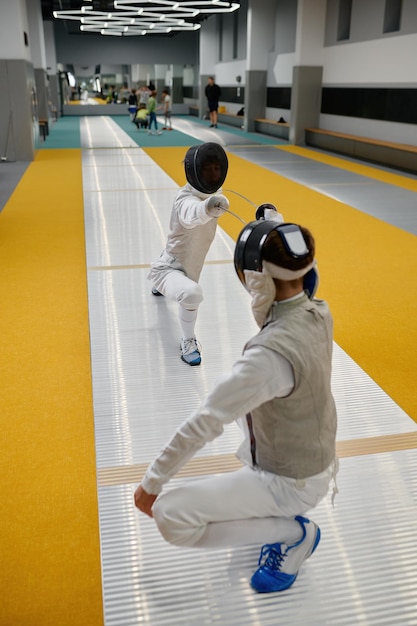In a brightly lit gymnasium, two fencers are captured mid-practice on an elongated, narrow path lined with a silver mat, reminiscent of a red carpet, but silver, laid over a mustard yellow floor. The surrounding area transitions between blue and yellow hues, suggesting a mix of flooring materials. Both athletes are donning traditional white uniforms, with protective black mesh helmets securely fastened. 

The fencer closest to the observer, seen from behind, is kneeling with one knee bent and the other perched on their toes, heels touching the ground. This individual is extending their fencing sword directly in front of them at head level, their left arm straight and aligned with their knee. Facing them, the second fencer is lunging forward with their right leg, aiming their sword at their opponent’s head, while their dark helmet partially reveals their determined visage. They each wear blue and silver tennis shoes, enhancing their mobility.

In the background, four other individuals are visible, one notably tall and clad in black shorts and a black long-sleeved shirt. The gymnasium's far end is bustling with onlookers and participants, highlighting the communal spirit of the sporting event. The intricacies of their movements are framed by the structured environment of the fencing area, with its distinct silver mats, yellow floor, and regimented lines, emphasizing the disciplined nature of this dueling sport.